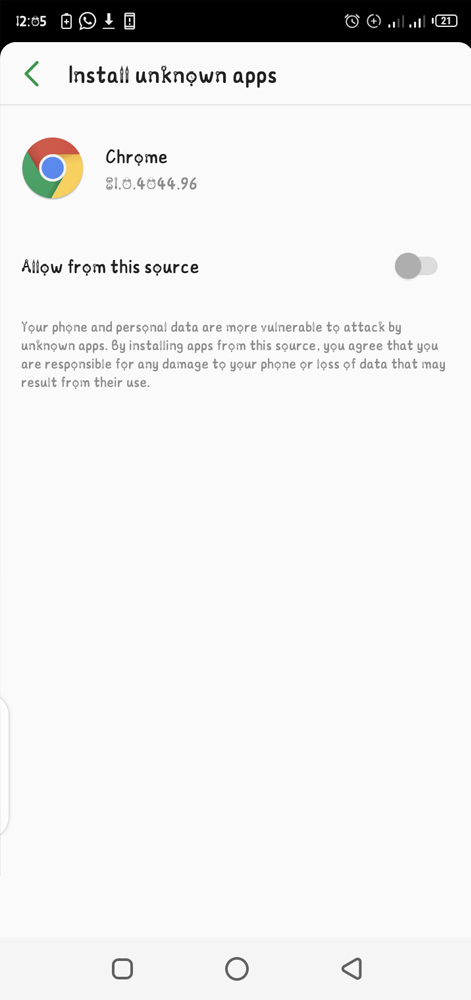The image appears to be a screenshot from a tablet device. In the upper left-hand corner of the screen, the time is displayed as 12:05, along with various icons: the battery icon showing 27% battery life, the download icon, and the alarm clock icon. 

Below this status bar, there is a green left-pointing arrow with text next to it saying "Install Unknown Apps." Directly beneath this text is the Chrome logo, characterized by a circle with segments colored red, yellow, and green, and a blue circle in the center. Next to the Chrome logo, it says "Chrome," and underneath it, there's a numerical value displayed as "104044.96."

Below this numerical value, there is text stating "Allow From This Source," which is highlighted with an error in spelling for "Source" (written as "S-Q-U-R-C-E"). Next to this phrase, there is a toggle switch currently set to the "off" position.

The final section of the image contains a warning message indicating that the user's phone and personal data may be more vulnerable to attack by installing unknown apps. The initial portion of the message is readable as "Tor phone and personal data are more vulnerable to attack by..."